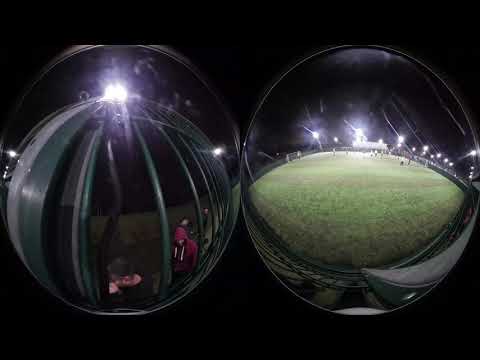The image depicts a nighttime outdoor event captured with a fisheye lens, giving it the appearance of two circular, orb-like views arranged horizontally like a figure 8. The left orb shows a scene framed by green slatted fencing with steel beams, lit by stadium lights. People are visible, including one wearing a black shirt and another in a red hooded sweatshirt, standing near the bottom center of this orb. The right orb offers a broader view of a well-lit soccer field with vibrant green grass, goalposts, and numerous bright lights surrounding the area. The background beyond the two orbs is solid black, emphasizing the bright, focused scenes within each circle-like view.